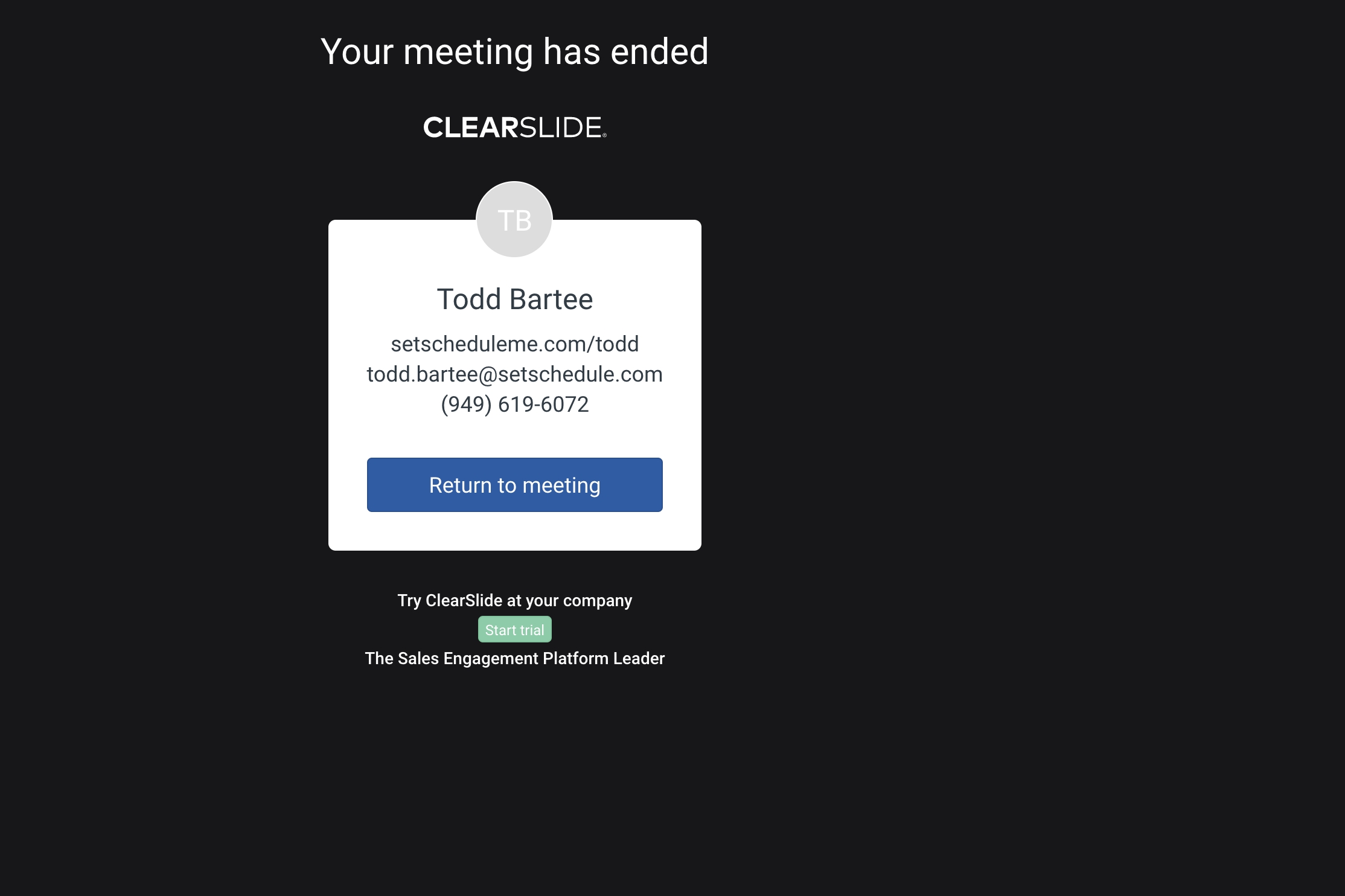The image has a black background with several elements arranged vertically. 

At the top, in white text on the black background, it reads "Your meeting has ended." Below this, another white text line reads "ClearSlide."

Central to the image is a white rectangle, within which a gray oval sits at the top, featuring the initials "TB" in its center. Directly beneath the oval, the following details are listed:
- Name: "Todd Bartee"
- Website: "setscheduleme.com/Todd"
- Email: "todd.bartee@setschedule.com"
- Phone number: "949-619-6072."

Below this information, there is a prominent blue rectangular button labeled "Return to meeting."

Further down, an invitation reads "Try ClearSlide at your company" in white text. Underneath this, a green button marked "Start Trial" invites interaction.

At the very bottom of the white rectangle, it states, "The Sales Engagement Platform Leader."

The remainder of the background is black, devoid of other elements.